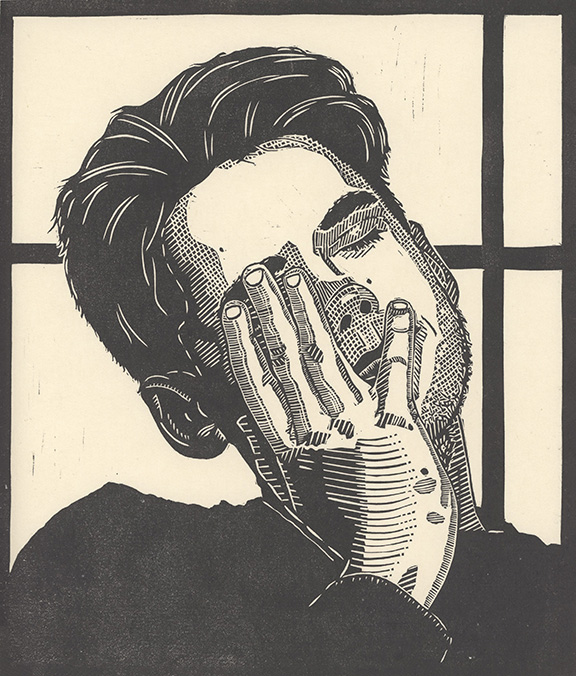The image is a detailed black and white drawing, likely done with black ink or paint on a white background that has a subtle pinkish tinge. It features a young adult man with short black hair, which is accented by some white streaks. His head is turned to the side, resting in his right hand, and he appears forlorn or frustrated, with his eyes closed. He is dressed in a black long-sleeved shirt, and the view captures him from above the head down to his chest.

The background is intricate with a series of lines and a window-like structure. There is a horizontal black line running left to right across his head and another line going vertically, meeting at his shoulder. Additional black lines cross the top, middle, and far right side of the image, resembling structural or window frame elements. The drawing includes black dots and sketch lines, particularly around the man's face and hand, adding to the texture and depth of the artwork. Despite the limited color palette and the sketch-like quality, there's a significant amount of detail, suggesting professional craftsmanship. The image is devoid of any text, focusing purely on the visual and emotional expression of the subject.